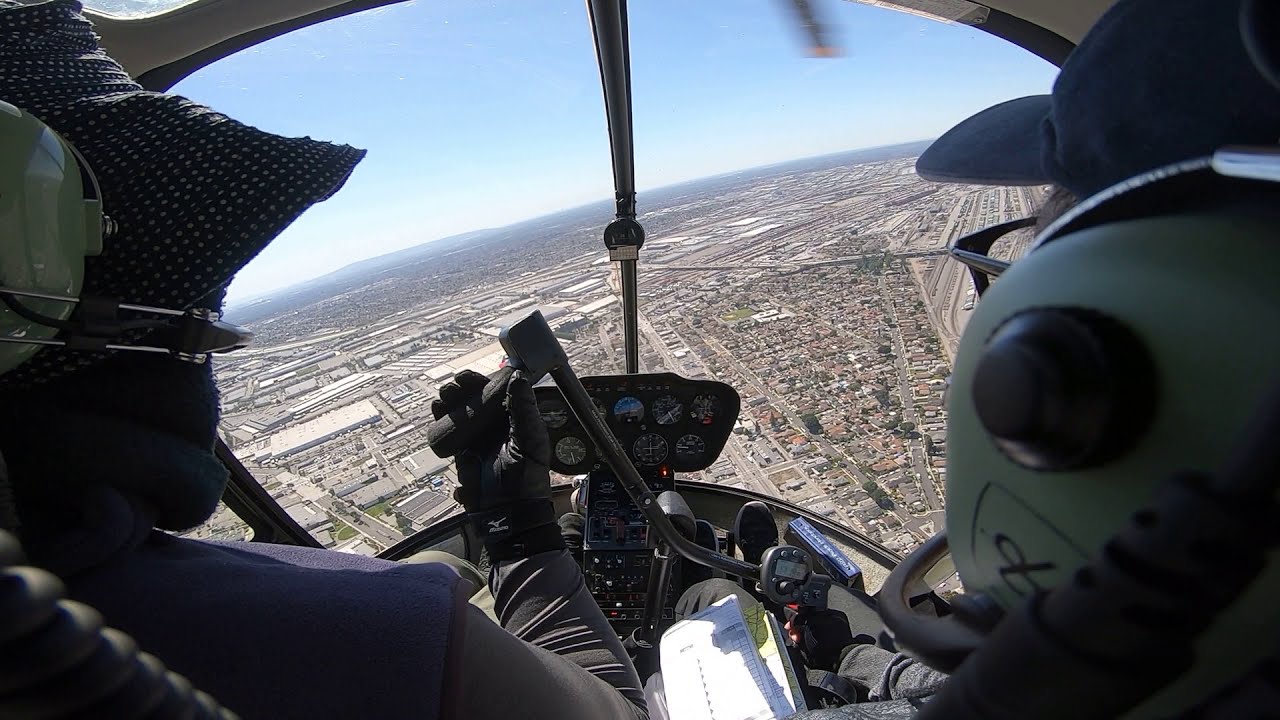The image captures the interior of a helicopter in mid-flight, providing a detailed view from behind the two front seats occupied by two individuals. Both individuals are wearing blue hats and green and black ear protector headphones for communication. The pilot on the right is holding the steering control stick, while the individual on the left, also handling a device with a grip, could be co-piloting or assisting. The control dashboard, predominantly black, is centrally positioned between them and slightly obscured by their seats.

Above the dashboard, the open sky extends in various shades of blue, contrasting with the cityscape below. The helicopter appears to be flying at a significant altitude, rendering the buildings and houses small. The urban area below displays a mix of residential and industrial zones, with visible red-tiled roofs and a large warehouse-like structure indicating the separation. The faint tip of the helicopter blade, colored red, is also faintly visible in the upper part of the image, adding to the detailed depiction of this aerial perspective. The entire scene subtly captures the blend of precision in the helicopter's cabin with the sprawling, varied landscape below.